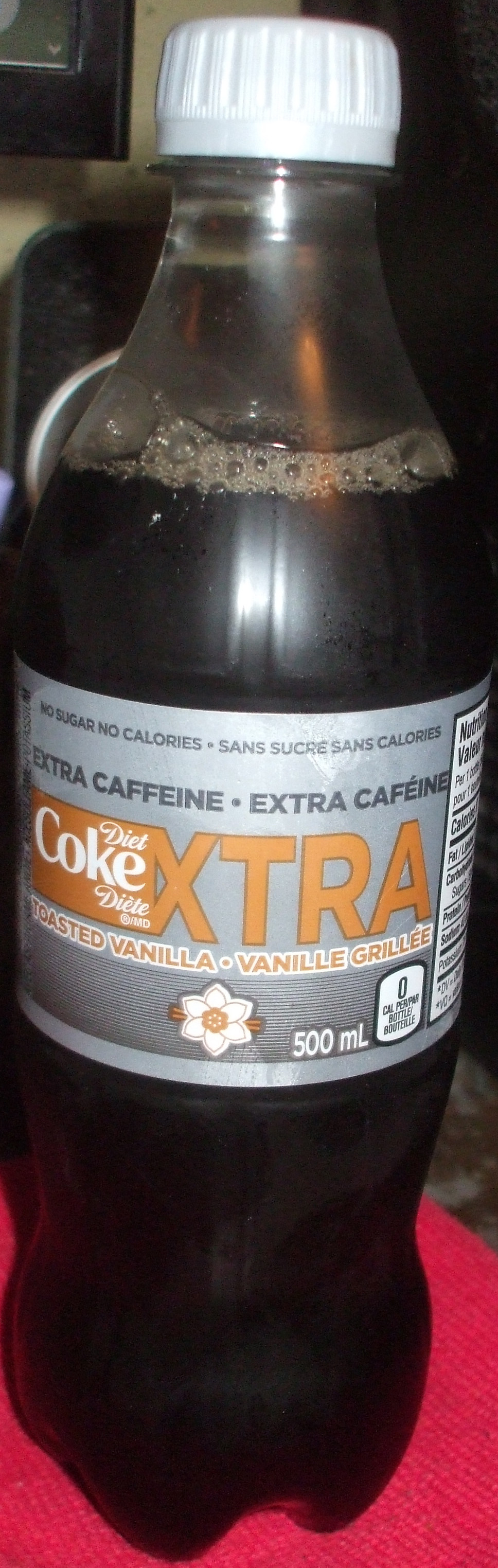A 500 milliliter plastic bottle of Diet Coke Extra sits on a red cloth. The bottle, sealed with a white cap, contains a dark brown liquid with foam on the top. The label, which is gray in color with orange and black lettering, features text in both English and French. Phrases such as "no sugar, no calories," "sans sucre, sans calories," "extra caffeine," and "extra caffeine A" indicate the product's characteristics. The label also mentions "toasted vanilla" and "vanilla grillé," emphasizing the flavor, and includes a picture of a vanilla flower. The right side of the label contains partially visible nutritional information. The product is branded as "Diet Coke," with an additional "diète" (D-I-E-T-E) to cater to bilingual consumers.